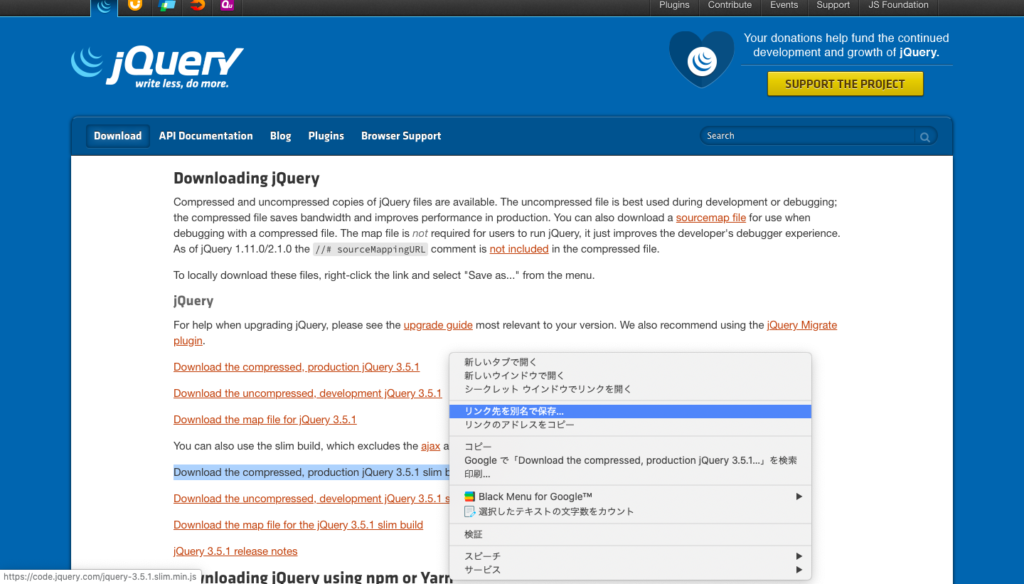This screenshot captures the homepage of the jQuery website. At the top of the page, there is a prominent banner that spans from left to right, featuring the jQuery logo alongside the tagline "jQuery: Write Less, Do More." To the right of the tagline, there is an icon resembling a heart and a message that reads, "Your donations help fund the continued development and growth of jQuery." Adjacent to this, a conspicuous yellow button labeled "Support the Project" encourages user contributions.

Beneath the banner, the navigation bar extends horizontally, listing several interactive buttons including "Download," "API Documentation," "Blog," "Plugins," and "Browser Support." To the far right of these buttons, there is a search field enabling users to quickly locate specific content or documentation on the site.

Further down the page, the section titled "Downloading jQuery" provides detailed information about the available jQuery files. It explains that both compressed and uncompressed versions of jQuery can be downloaded. The uncompressed file is recommended for development and debugging purposes due to its readability, while the compressed file is optimized for production use as it conserves bandwidth and enhances performance. Additionally, the site offers a source map file for debugging compressed files, although it points out that the map file is not necessary for running jQuery.